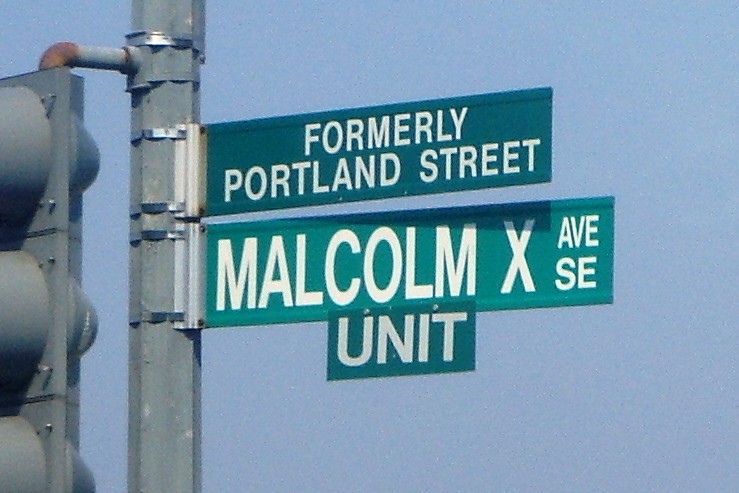In this highly magnified and slightly grainy image, the focal point is a series of street signs against a backdrop of a clear, light blue sky. Dominating the left side of the frame is a sturdy, gray metal pole standing upright. Attached to this pole, there's a standard gray traffic light, whose cylindrical sections are aligned vertically in anticipation of displaying the usual sequence of red, yellow, and green lights.

Extending horizontally from the right side of the pole are two green street signs with crisp white lettering. The upper sign reads "Formerly Portland Street" while directly below it, the second sign is labeled "Malcolm X Ave SE". Adding to the clarity and detail, a smaller rectangular placard is firmly affixed at the center of the lower sign, bearing the label "unit." This setup of signs, articulated against the serene sky, not only directs traffic but also narrates a piece of the locale's history and commemoration.